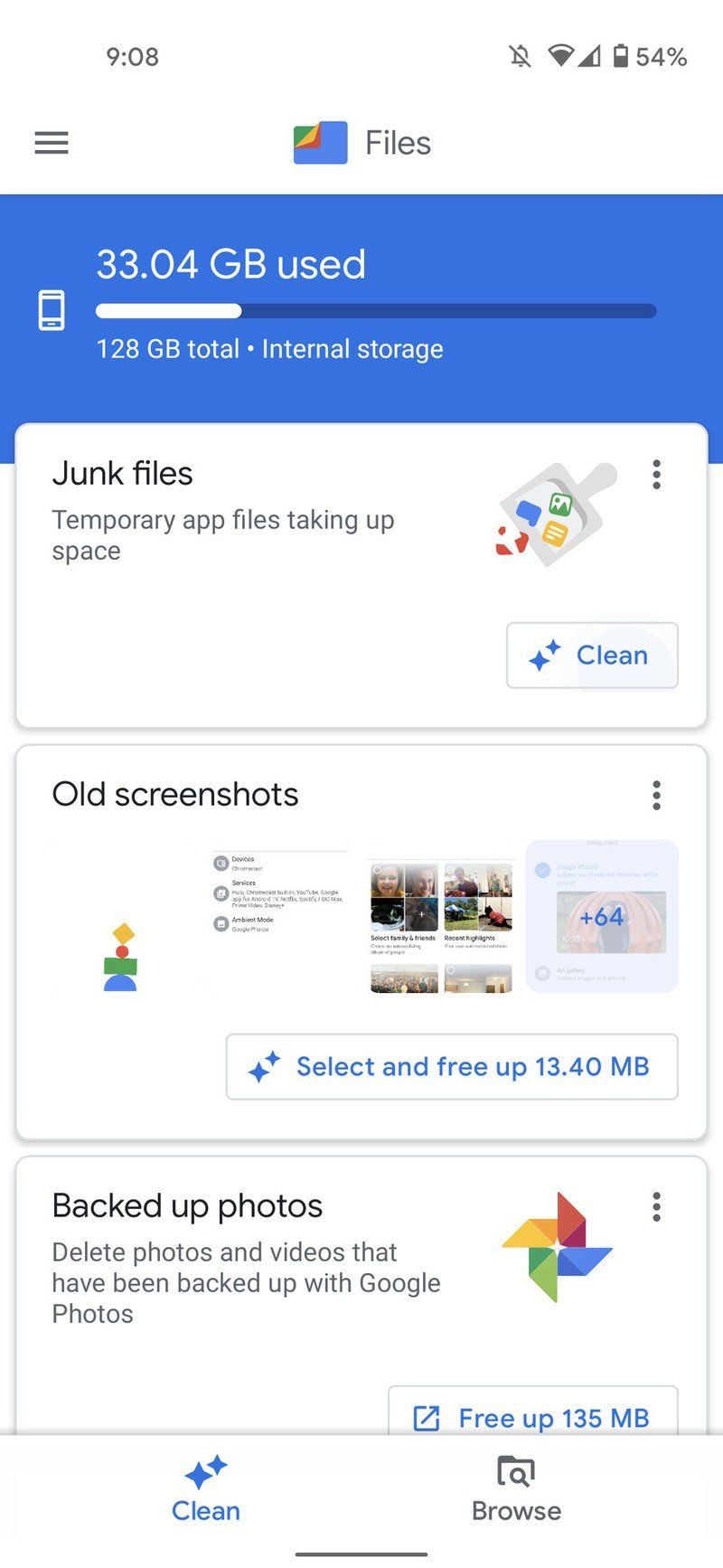In this smartphone screenshot, the time displayed at the top of the screen is 9:08 AM. The status bar also shows essential icons: the battery icon with its percentage, network connectivity, and WiFi signal strength. The "Files" app is open, characterized by a black, three-line icon on the top left corner for options.

A blue bar prominently details the phone's storage usage, indicating that 33.04 GB out of a total of 128 GB is currently used. The text within the bar is elegantly formatted in white against the blue background for clear visibility.

Below the storage summary, a section highlights "Junk files" and "Temporary app files taking up space," written in black text on a white background. An icon resembling a trash can accompanies this text, followed by a "Clean" button for action.

Further down, another white band is labeled "All screenshots," providing an option to clean up the screenshots on the device. Similarly, there is a section for "Backup photos," also with a cleaning option. The caption "Clean" and "Browse" options are visible, guiding the user through the file management process.